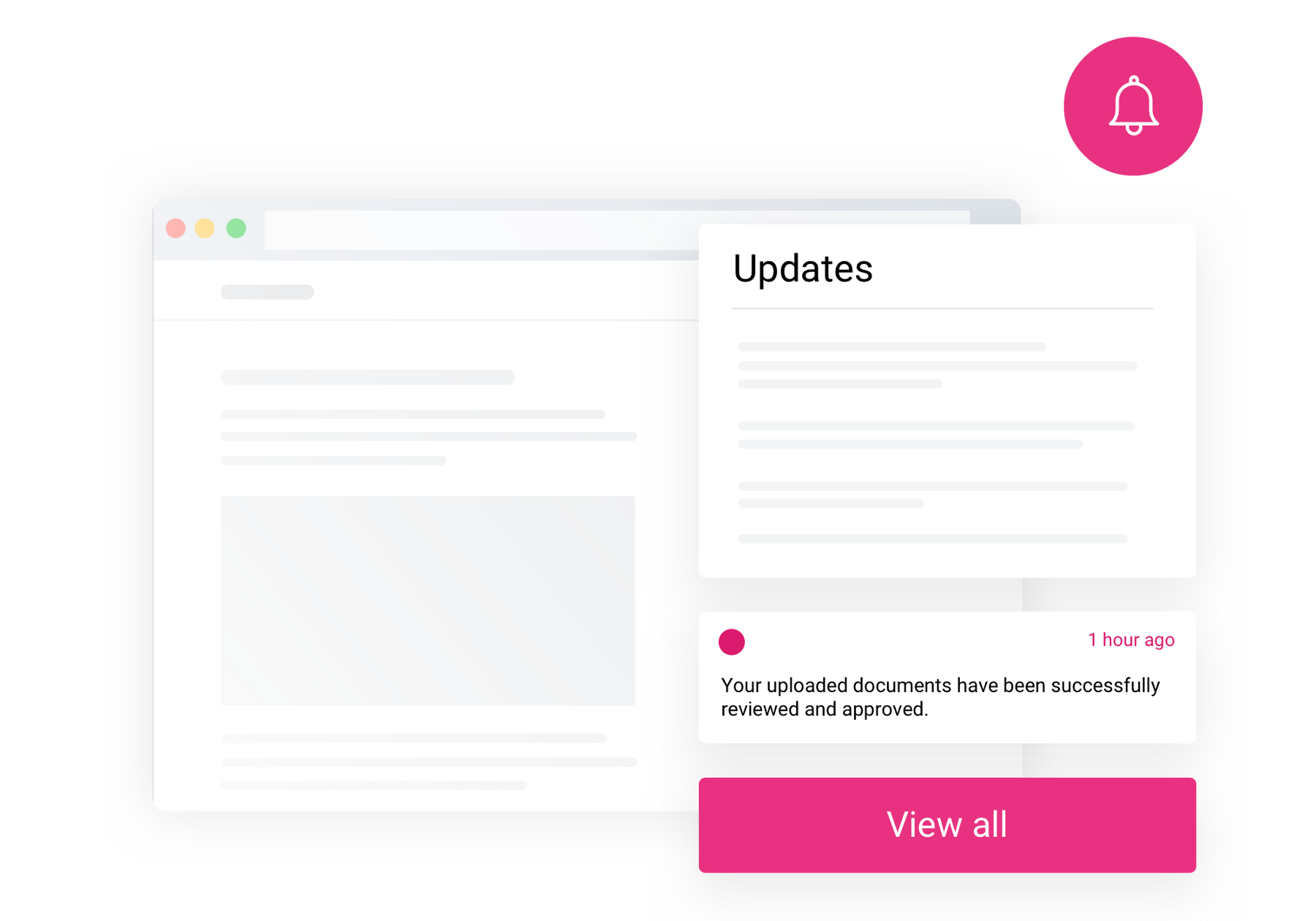The image depicts a webpage with a basic outline of a web browser in the background. At the top, there is an empty, white search bar framed in medium light gray. The main section features several light gray lines and boxes, suggesting placeholders for text and images. 

In the upper right corner of the page, a large hot pink circle contains a white bell-shaped icon, indicating notifications. Directly below is a white square superimposed over the background, with a black heading titled "Updates." Underneath this heading, there are several light gray bars representing lines of text within the white box.

Further down on the right, another white box contains a small bright pink dot in the upper left corner. Opposite the dot, on the upper right, is pink text that reads "one hour ago." Below this timestamp, black text states, "Your uploaded documents have been successfully reviewed and approved." Further down is a prominent hot pink rectangular button with large white text that reads "View All."